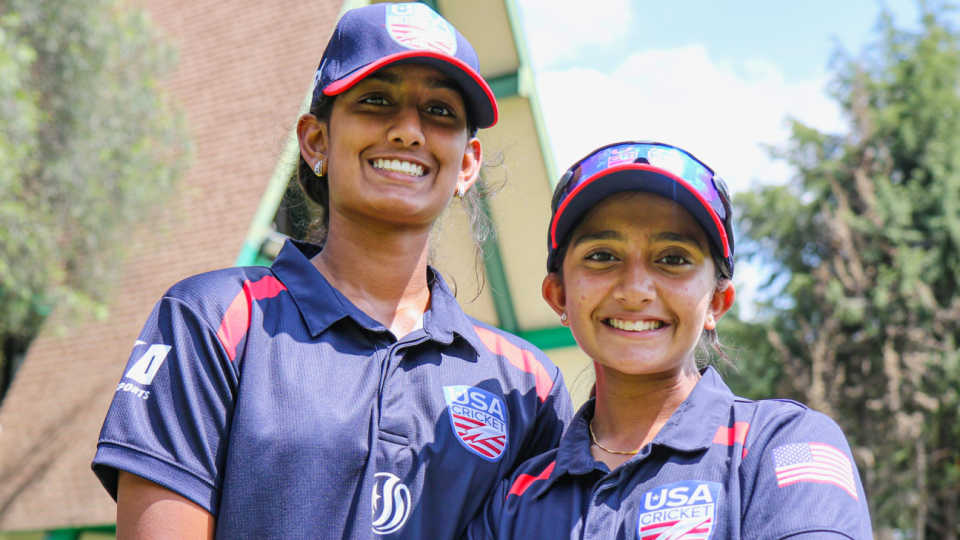This image features two young Indian or possibly Middle Eastern women standing outdoors, smiling directly at the camera. They are dressed in matching navy blue collared polo shirts emblazoned with the USA Cricket logo inside a shield, an American flag on the right shoulder, and red stripes near the shoulders. Both women are also donning navy blue baseball caps with red brims and the same USA Cricket logo at the front. The woman on the right is slightly shorter, wearing glasses perched atop her cap, and a gold chain necklace, along with small stud earrings. The woman on the left is taller, adorned with black and white earrings. Their hair is pulled back, revealing their medium to dark complexions and dark eyes. 

In the background, there is an A-frame house painted white with green trim and a shingled roof. The scene also includes a bright blue sky filled with some puffy white clouds and flanked by trees on both the left and right sides of the frame. The overall mood is cheerful and vibrant, capturing the essence of camaraderie and team spirit.